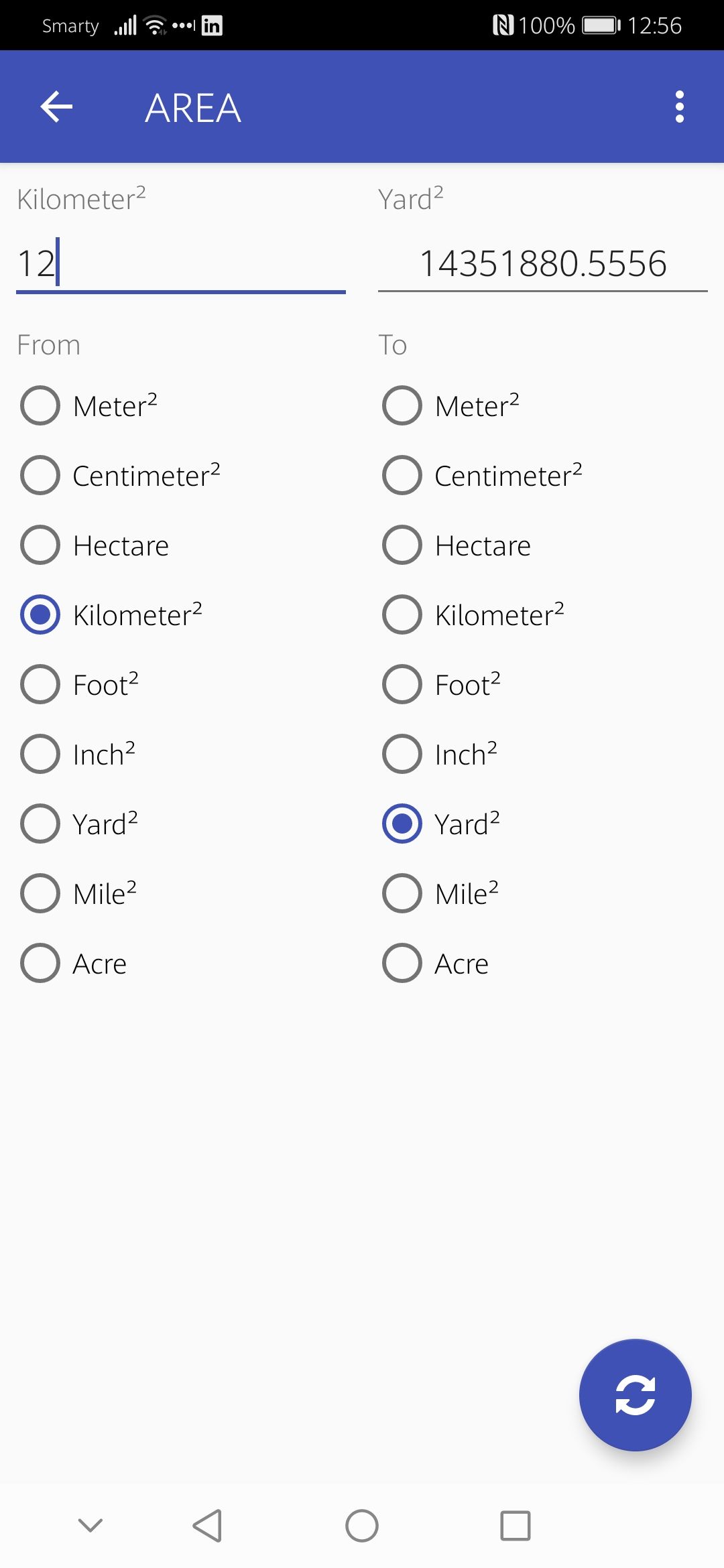This image is a detailed screenshot of a conversion app designed to translate between metric and standard measurements. At the top of the screen, the user's status icons are displayed, indicating full cell signal, Wi-Fi connection, a 100% battery level, and the time, which is 12:56. Three white dots in the upper-right corner provide an option to access additional information or settings within the app.

Below these indicators, a prominent blue bar labeled "Area" signifies the category of measurement being converted. The app interface is divided into two main columns with a clean white background. The left column is labeled "Kilometer" and the right column is labeled "Yard." Users can input a value in kilometers to convert it into yards. 

The app offers a versatile selection of units for conversion; users can choose between meter, centimeter, kilometer, foot, inch, yard, mile, and acre from the left column, and convert them to yard, inch, foot, kilometer, centimeter, or meter in the right column. 

A refresh button featuring circular traveling arrows is located at the bottom of the screen, providing a quick way to reset the input fields for new conversions.